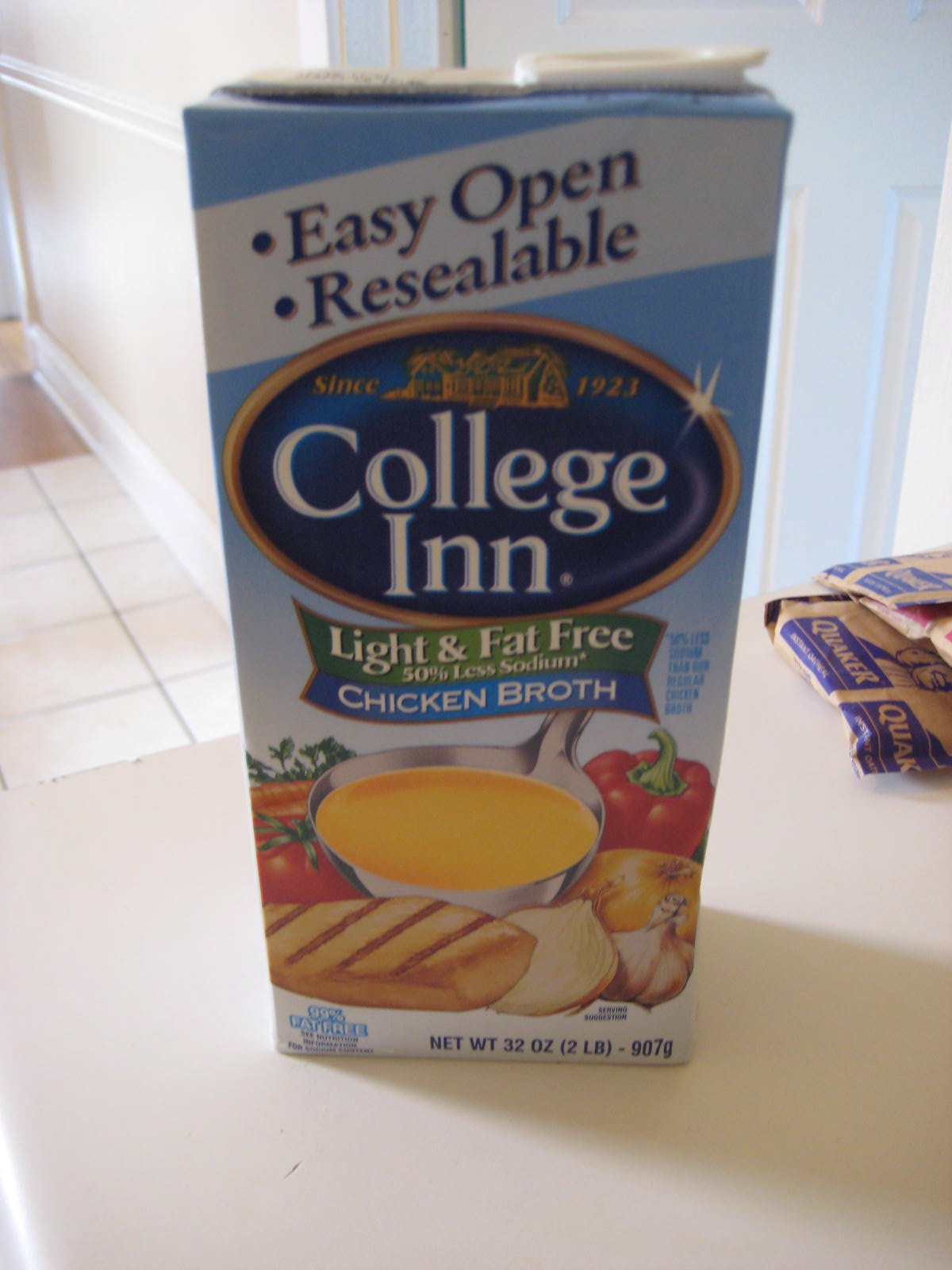The photograph, captured in a kitchen, prominently features a carton of College Inn light and fat-free, 50% less sodium chicken broth sitting on a smooth white tabletop. The wall behind the kitchen is plain white, and the floor is adorned with white square tiles. To the right of the chicken broth carton, partially cut off by the edge of the image, are three Quaker oatmeal packets in distinctive colored prints—purple, blue, and red, indicating different flavors.

The College Inn chicken broth carton is primarily light blue at the top, fading into white, and adorned with a colorful array of vegetables at the bottom, which includes capsicum, onions, tomatoes, and a cut of meat. It features a silver tone pot filled with orange broth on the front. A white diagonal banner across the top states "Easy Open Resealable," accompanied by a blue dot. Underneath, a golden oval border houses the words "Since 1923" and a graphic of an inn, followed by "College Inn" in white lettering. Below this, in green and blue banners with white letters, it reads "Light and Fat-Free, 50% Less Sodium" and "Chicken Broth." The net weight is noted at the bottom right as 907 grams, 2 lbs, 32 oz. The image is likely taken vertically on a phone, emphasizing the rectangular shape of the carton.